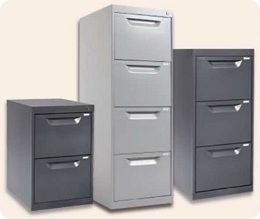The image depicts three metal filing cabinets set against a tan or off-white background, possibly part of an office supply catalog. Each cabinet is slightly angled, presenting a partial side view. From left to right, the cabinets vary in size and color. The cabinet on the left is black, the smallest of the three, with two drawers. The middle cabinet is gray and the largest, featuring four drawers. The rightmost cabinet is black with three drawers and is the second tallest. Each cabinet includes a keyhole located in the upper right corner of the top drawer. The drawers lack protruding handles and instead have recessed pulls, allowing users to pull them open with their fingers from underneath. The image shows that the cabinets are almost as deep as they are wide.